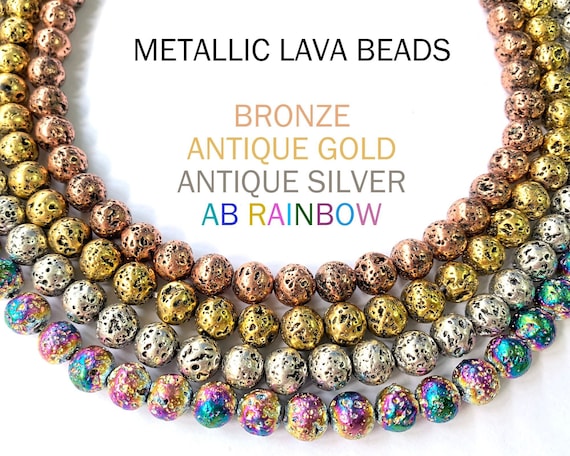The image displays a detailed, close-up view of four semicircular rows of textured beads arranged in a U-shape against a white background. The beads feature distinct textures with grooves and pits, lending a tactile quality. Centrally, black text announces "Metallic Lava Beads," followed by categorically colored labels for each row: "Bronze," "Antique Gold," "Antique Silver," and "AB Rainbow." Each corresponding row showcases the labeled color; bronze beads form the first row, antique gold beads the second, antique silver beads the third, and the iridescent AB rainbow beads the fourth. The rainbow beads exhibit a mesmerizing array of colors, including aqua blue, yellow, pink, green, indigo, and lilac, reminiscent of an oil slick’s shimmering hues. The overall composition of the beads is reminiscent of a cascading necklace, creating an elegant and visually dynamic pattern.